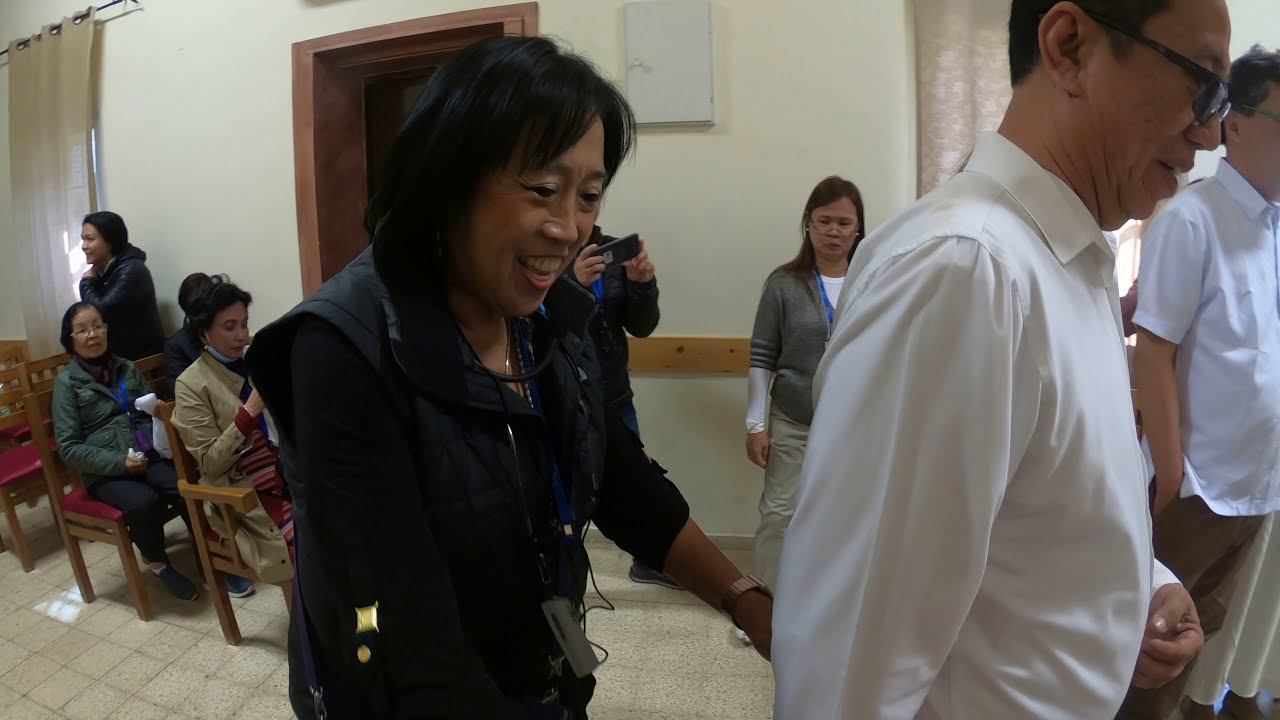In an indoor setting, a photograph captures a seemingly ceremonial or formal event. At the forefront stands an older Asian man with black hair wearing dark sunglasses or glasses and a white long-sleeved button-up shirt; his head is slightly tilted down, giving him multiple chins. Standing close behind him is an older Asian woman with chin-length black hair, a centered parted fringe, and adorned in a black vest over a long-sleeved black shirt, which has a distinct gold accent on one arm. She smiles widely and extends her left arm forward, seemingly holding onto the man's shirt. To their right, slightly in the background, appears a man mostly cropped out of the photo, dressed in a short-sleeved white collared shirt and brown pants, hands tucked into his pockets. The setting is completed with light-colored linoleum flooring and a pale white wall, against which some brown wooden chairs are aligned; these chairs are occupied by sharply dressed people, mostly wearing white shirts, with one woman visible in the scene wearing a blue lanyard. In the far background, a person is seen taking a photograph with a cell phone.